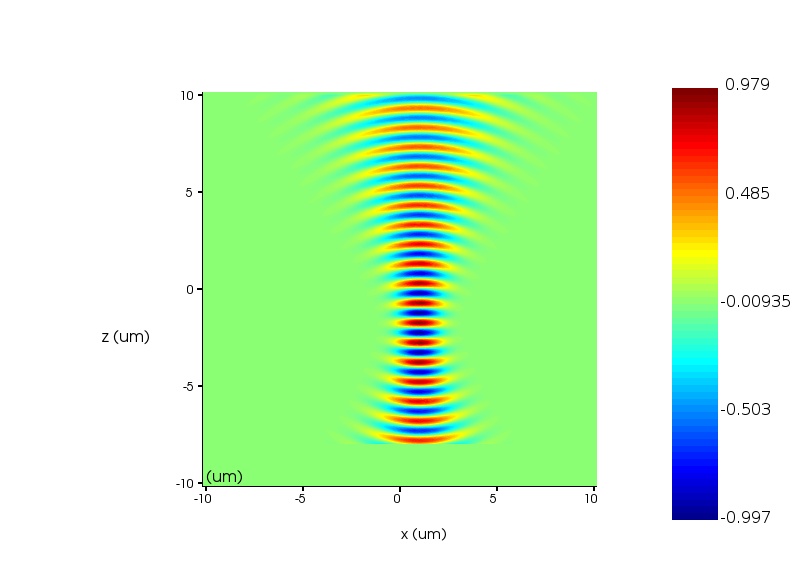The image depicts a highly vivid and detailed digital screenshot of a meter spectrum. To the right, there is a vertically positioned, neon-colored bar chart with a gradient transitioning from deep red through various shades of orange, gold, yellow, lime green, mint green, aqua blue, tropical blue, cobalt blue, to deep Mediterranean blue. This bar ranges in values from 0.979 at the top to -0.997 at the bottom. Adjacent to this bar, approximately an inch away, is a green square plotting chart with horizontal and vertical demarcations. The Y-axis values range from -10 to 10, and the X-axis mirrors this range.

Within the center of the square chart, there are radiating arcs colored in yellow, blue, orange, lighter blue, and cobalt blue. These arcs give the appearance of inverted bowling pins and display a seemingly dynamic spin effect due to the way they are presented. The chart background is a heavy neon green, making it quite striking and somewhat overwhelming to view with its intense brightness. The details include slashes of red, blue, and yellow colors intersecting the middle of the axis, contributing to the image's overall vivid and neon-like aesthetic. The axes are labeled 'Z of nanometers' and 'X of nanometers,' reflecting the spectrum's measurement in nanometers.